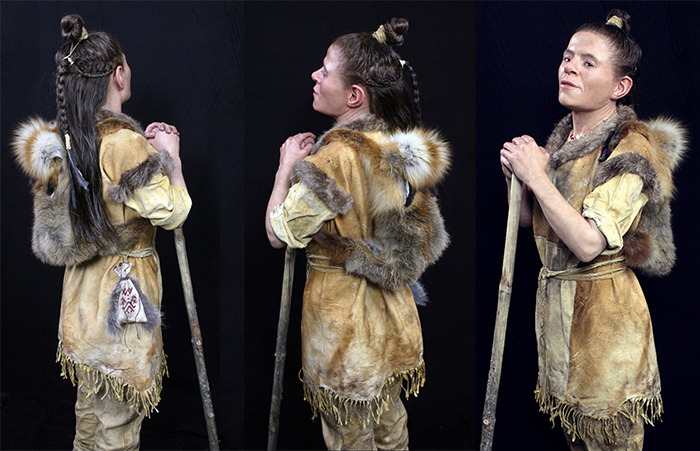The image consists of three photographs capturing a detailed portrayal of a fair-skinned woman with dark brown hair styled in a unique manner—half tied up in a bun with two smaller braids merging into a large braid down her back, while the rest of her hair flows straight. She is depicted wearing a tribal animal skin coat, tan in color with a mix of dark brown, medium brown, and white fur on the back. The ensemble includes off-white trousers and a tan long shirt jacket adorned with fringe. Each photo, showing different angles, highlights her holding a long walking stick and a small white pouch adorned with red symbols and fur accents hanging from her shoulder. Two photos capture her from variations of her back and sides, while the third shows her front and profile, offering a comprehensive view of her attire and accessories, including a necklace. The woman's serene expression underscores the overall tribal and prehistoric aesthetic of the scene.